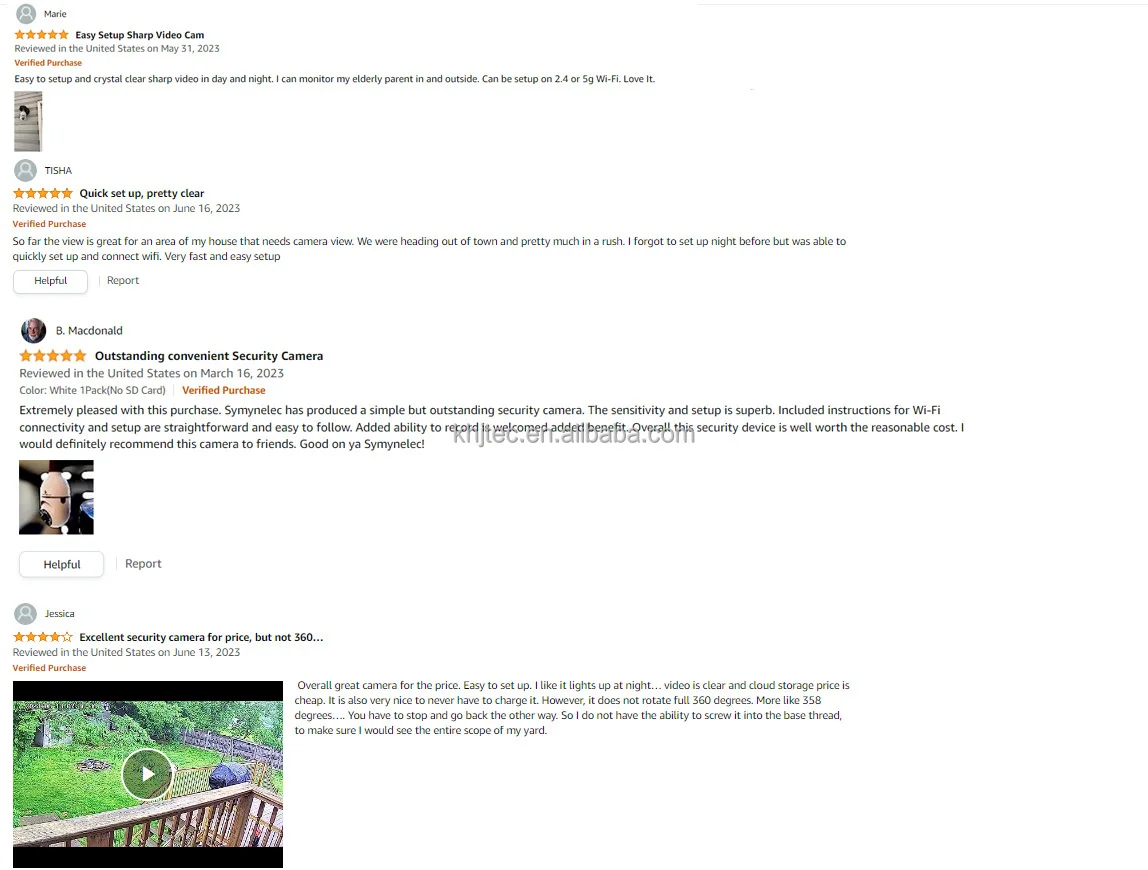This image, captured from a computer screen, displays customer reviews for a "Sharp Video Camera" product, potentially from Amazon or a similar retail site. The page header mentions the camera's name prominently. Each review has a "Verified Purchase" badge in orange, confirming authenticity. 

The first review praises the camera's ease of setup and its crystal-clear, sharp video quality both day and night, mentioning its usefulness for monitoring an elderly parent both indoors and outdoors. The reviewer also notes the camera's compatibility with both 2.4 GHz and 5 GHz Wi-Fi bands, expressing overall satisfaction with "love it." Unfortunately, the star rating for this review is obscured by an unknown element on the screen.

The second review, written by Tisha on June 16th, 2023, describes a "quick setup" and "pretty clear" video quality. Tisha appreciates the wide coverage for a critical area of her house. Despite being in a hurry to leave town, she was able to set up and connect the camera to Wi-Fi promptly, remarking on the speedy and user-friendly installation process.

Below each review, there are interactive buttons where users can mark the review as "helpful" or "report" it. Additionally, two more reviews are partially visible towards the bottom of the image.